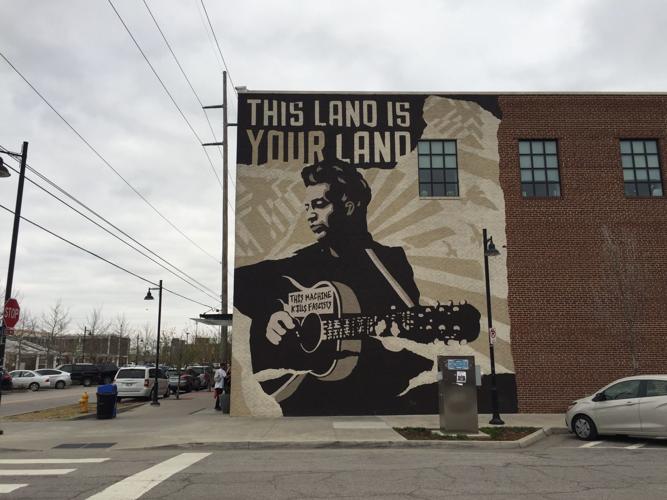The horizontally oriented, rectangular image, wider than it is tall, captures an outdoor urban scene under a cloudy, light gray sky. The central focus is a brick building adorned with a large mural. The mural, occupying a significant portion on the left side of the building, features an African American man dressed in black, strumming a guitar. Written on the guitar is the phrase “This machine kills fascists,” and above the mural, in a black background with white lettering, is the phrase “This land is your land.” The building's second floor has three blue windows with bars or brown squares covering them.

In the foreground, a tan car is parked to the right, adjacent to a metal utility box with several signs on it. To the left of the brick building is a street running alongside it, populated with several parked cars and a person standing nearby. The streets are lined with sidewalks and include various urban elements such as a yellow fire hydrant, a blue mailbox, and a few 20 to 30-foot tall utility poles with electric wires overhead. Additional visible details include a stop sign and street lights at various points, contributing to the realistic and bustling cityscape depicted in the photograph.